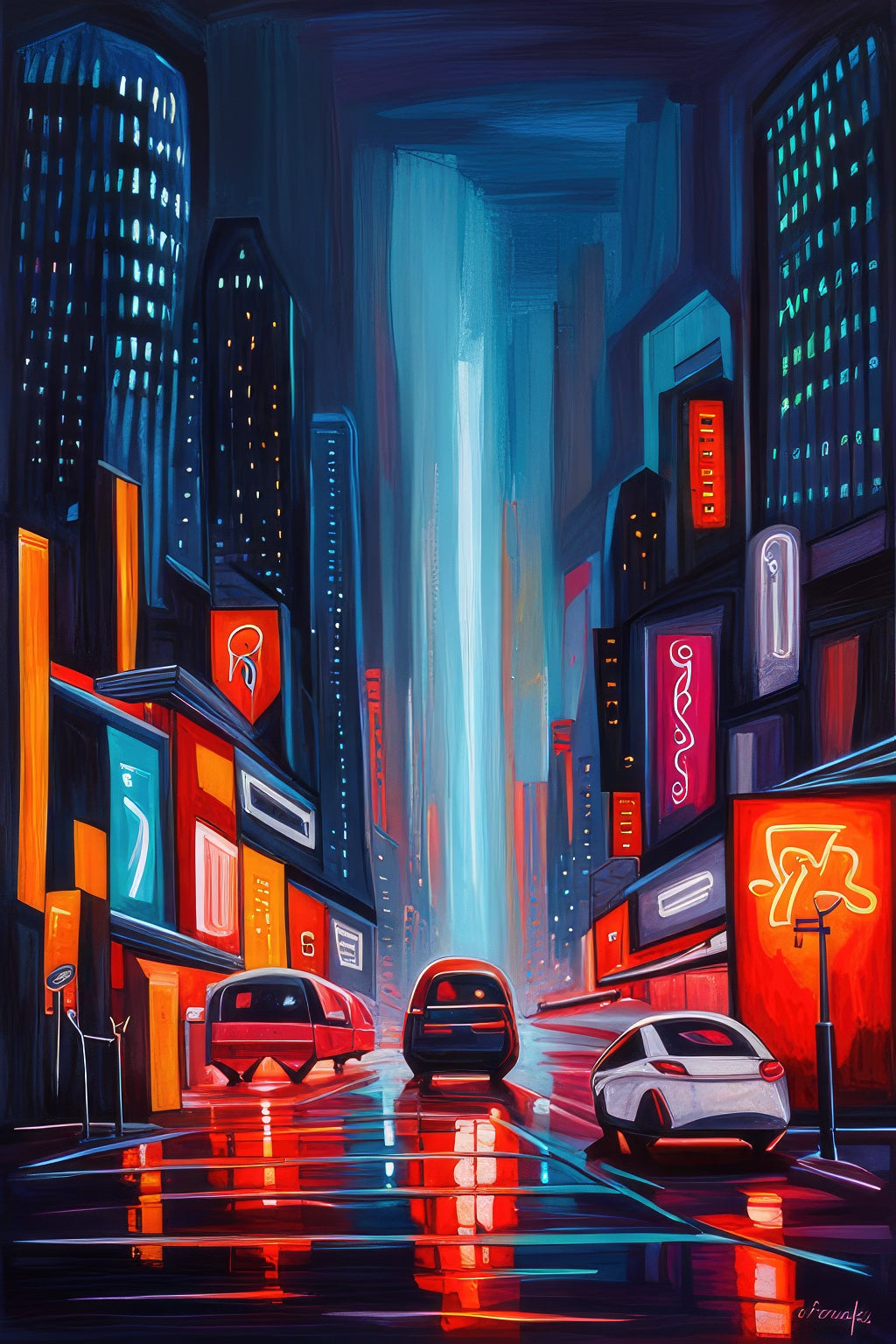"An animated poster with a minimalist aesthetic captures an evening cityscape. The sky, enveloped in a dark blue hue, sets a nighttime ambiance. Flanking the scene, buildings on both the left and right sides are depicted in various shades of blue, accented by simplistic green, light blue, and yellow squares symbolizing illuminated windows. Despite the lack of intricate details like window bars, the presence of these lights conveys a bustling urban environment. Below, a sleek, rain-slicked road reflects the subtle glow of the surroundings. Three vehicles occupy the street; on the right is a white car, while the central and left lanes feature gray and orange cars, all rendered without fine details, emphasizing the minimalistic design."